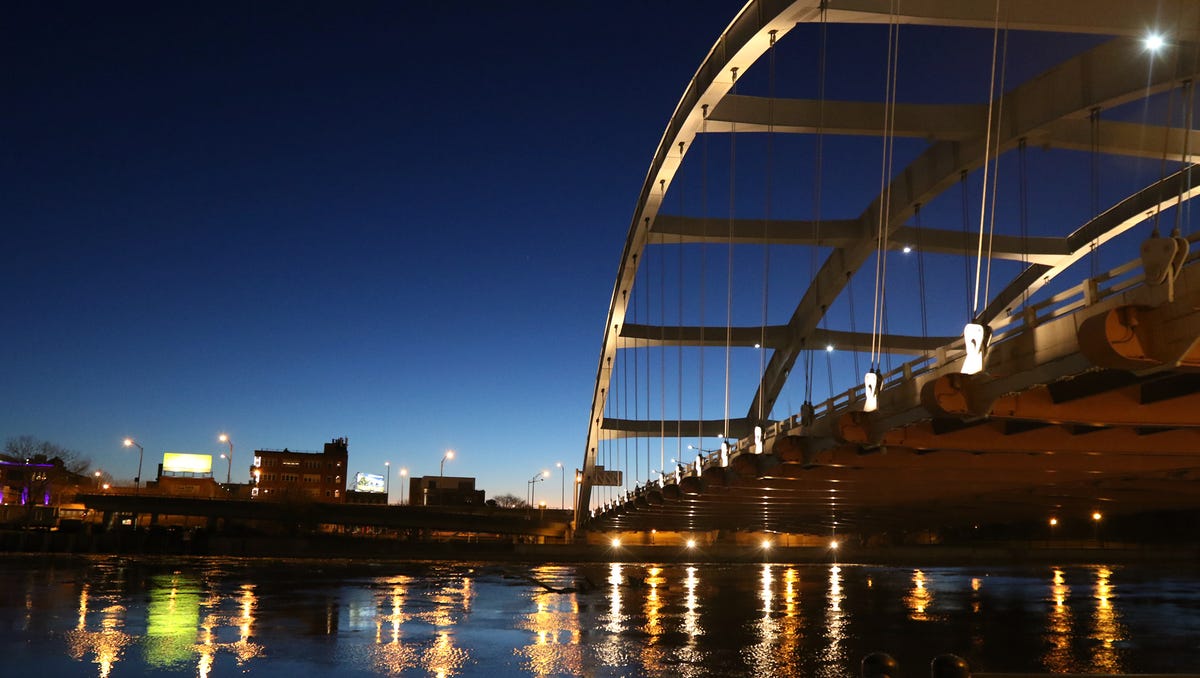A rectangular photograph captures a serene night scene with a balanced composition and striking details. In the right section of the image stands a prominent suspension bridge, characterized by a large golden metal archway that towers over the bridge deck. This bridge features concrete railings on either side and is illuminated by white lights hanging down from wires, casting a captivating reflection on the smooth, dark surface of the river below. The water's mirrored surface also captures yellow lights from beneath the bridge and various reflections from across the shore.

The top half of the photograph is dominated by an early evening sky, transitioning from dark blue at the very top to a lighter blue gradient towards the middle, suggesting a recent sunset. On the left side, the distant shoreline is dotted with the silhouettes of commercial buildings and billboards. Notably, there is a green billboard and buildings adorned with purple lights. A tall structure, potentially a parking garage, and a large illuminated building with a bluish hue are also visible amidst the array of urban elements. The overall composition effectively combines natural and artificial elements, creating an atmospheric and detailed nightscape.